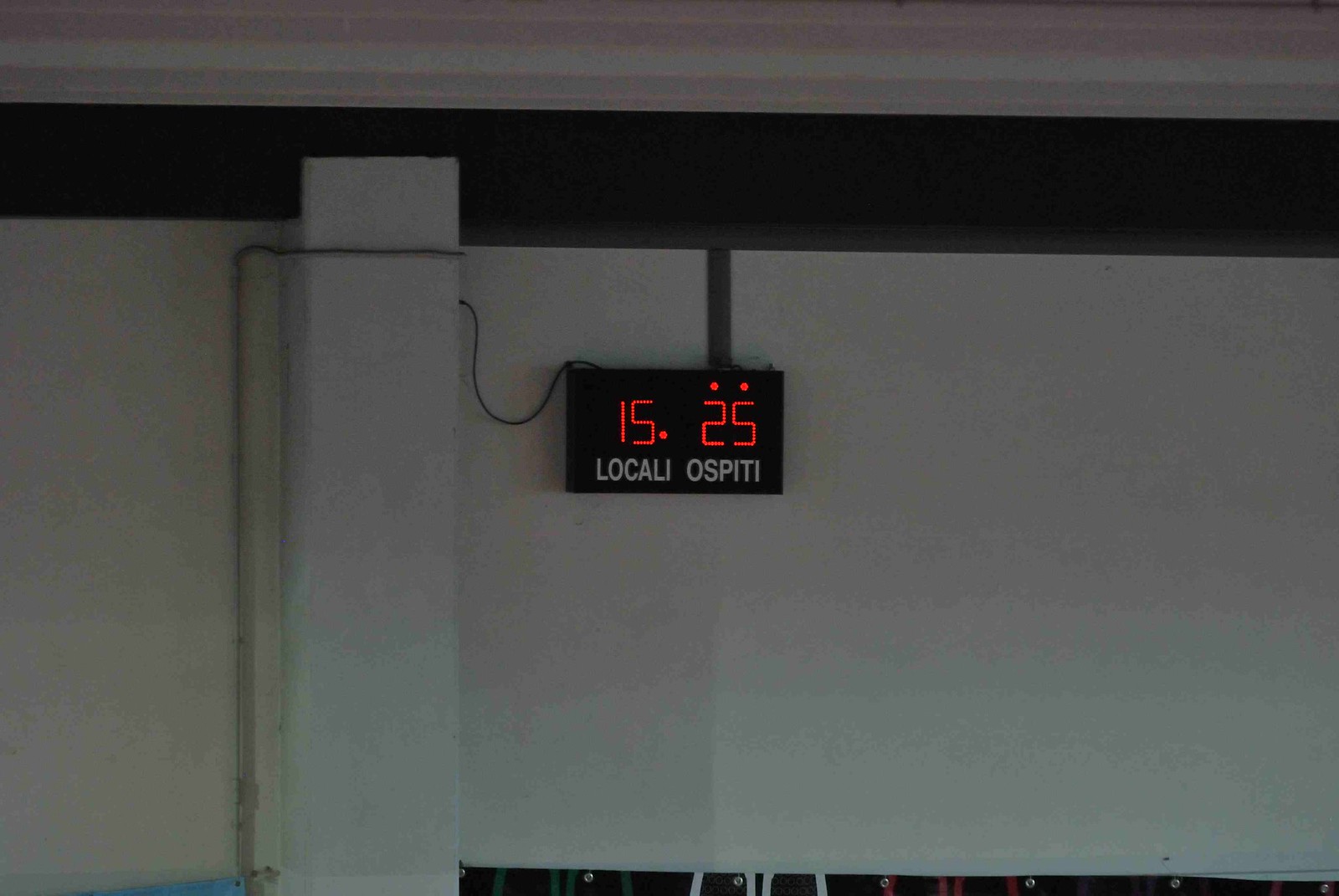The image captures a section of a white wall featuring a prominent black molding at the top. From this molding, a neon sign is suspended. The sign displays the words "Locali Ospiti" in white letters, divided into two lines - "Locali" on the top line and "Ospiti" on the bottom line. Above the word "Locali," the number "15" in red neon lights appears, and above "Ospiti," the number "25" similarly glows in red. Next to this, there is a black box or panel from which a cord extends, running down the wall before disappearing into it. The photo also includes a snippet of the ceiling, which is gray, adding to the overall contrast seen between the black, white, and red elements. The black molding, which frames the top of the wall, runs horizontally across. The combination of the sign and cord suggests a possibly electronic display, perhaps a digital clock or some form of informational display panel.